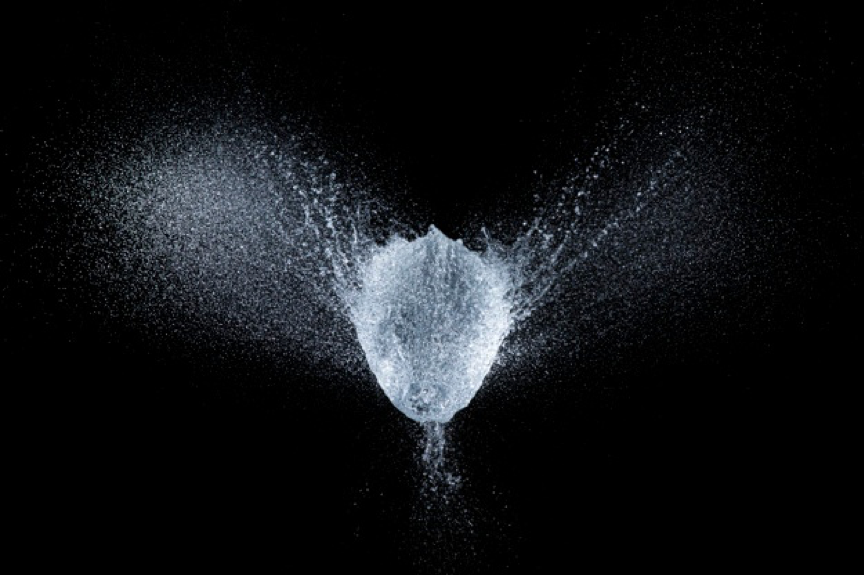This striking black and white photograph captures water mid-splash against a stark, pitch-black background, offering a highly detailed and dramatic scene. At the center of the image, water appears to be falling and spinning, forming a funnel-like shape, with droplets splashing outward on either side. The distribution of droplets is uneven, with more visible on the left-hand side than the right. The water, a clear whitish color, creates the illusion of an angelic figure with wings, as the splashes on both sides resemble outspread wings against the darkness. The close-up nature of the photograph enhances the abstract beauty of the splashing water, making it look almost like an ethereal entity suspended in mid-air.